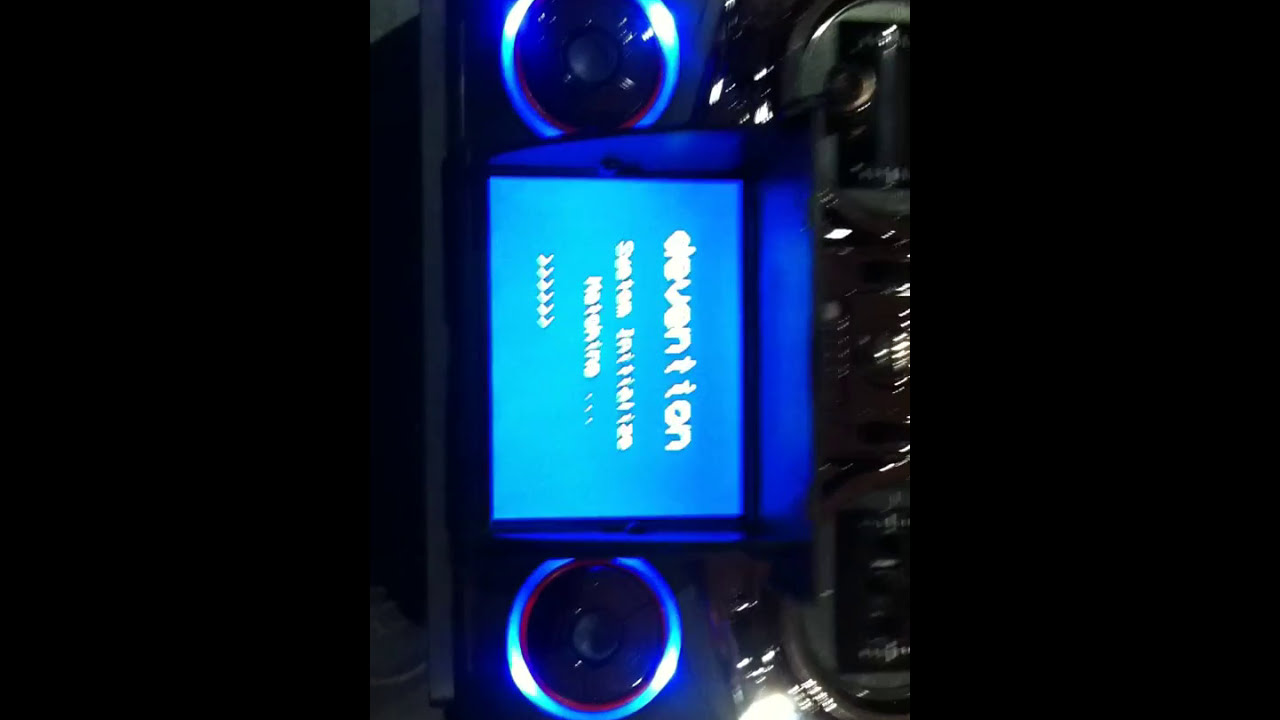In this rotated photograph, an electronic device rests at the center, highlighted by a vibrant blue glow. Dominating the device is a display screen with a blue background, displaying unreadable white text. Flanking the screen, two circular elements emit blue light, suggesting the presence of speakers. The orientation is shifted 90 degrees clockwise, adding to the confusion. The image itself is blurred, making specific details difficult to discern. On both sides of the device are thick black vertical strips. Additional features include silver-bordered circles, possibly dials, and a prominent light source at the bottom, casting a bright, albeit limited, illumination. The overall composition includes sporadic, indistinctly lit elements, contributing to a shiny, out-of-focus visual experience.